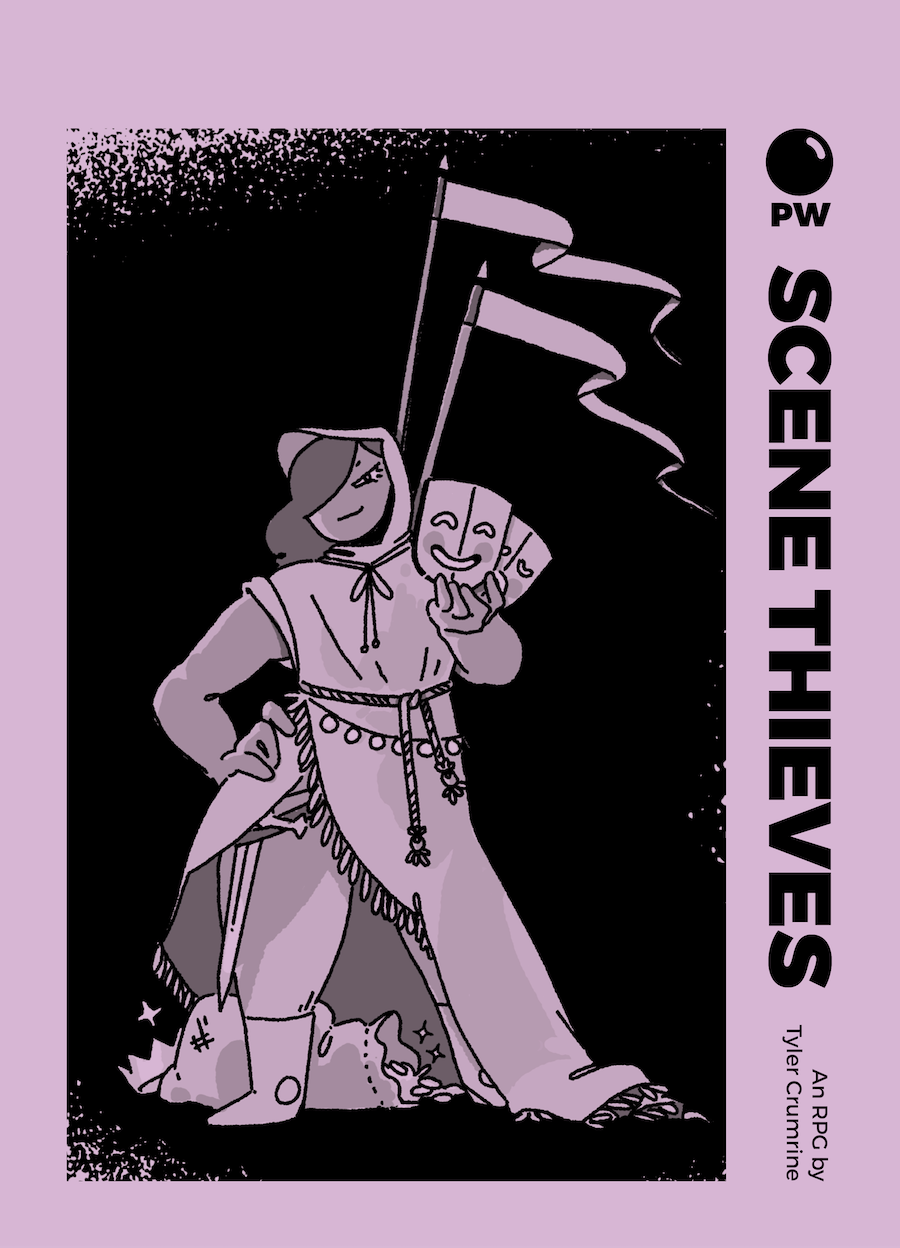This image is an advertisement, possibly for a play or a game, featuring a striking black and purple color scheme. The left side showcases a detailed illustration of a female character clad in medieval garb, complete with a cloak, boots, and a knife strapped to her leg, indicating she is a warrior. She holds two theater masks, one smiling and one frowning, in her hands. Purple flags are positioned behind her, adding to the dramatic atmosphere. The background of the left side is primarily black with a splash of light illuminating the upper left corner, enhancing the character's prominence. On the right side, in vertical text, the title "Scene Thieves" is displayed, preceded by the logo "PW" near the top. A smaller text beneath the title reads "an RPG by Tyler Kameeran," suggesting a connection to a role-playing game. The overall design is reminiscent of a band poster, emphasizing its promotional intent.